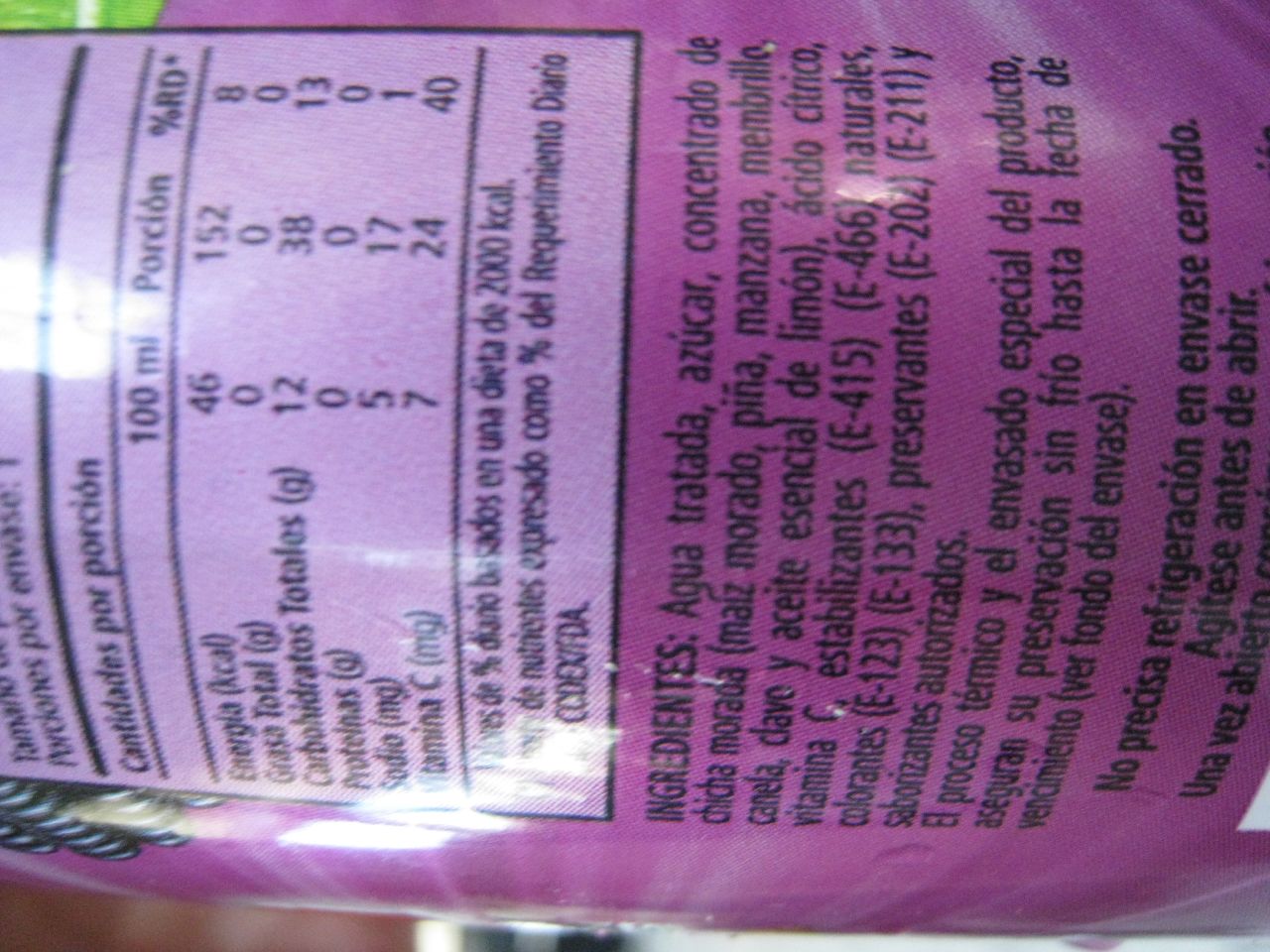The image is a close-up of a label on a possibly round food container, featuring a prominently curved surface. The container itself is a vibrant dark pinkish-purple with light violet stripes. The label's background alternates between lighter and darker shades of purple, with black text printed throughout. The upper portion of the visible label showcases the bottom part of a nutrition facts section, framed in a black outline box with a light purple background. The text includes nutritional information written in Spanish, such as ENERGIA 46, GRASIA total 0, CARBOHIDRATOS total 12, PROTEINAS 0, SODIO 5, and VITAMINAC with corresponding numerical values. There is some glare, possibly from flash or lighting, that distorts portions of the text. Below the nutritional section, within the darker purple area, is the ingredients list, also in Spanish, printed in black writing.